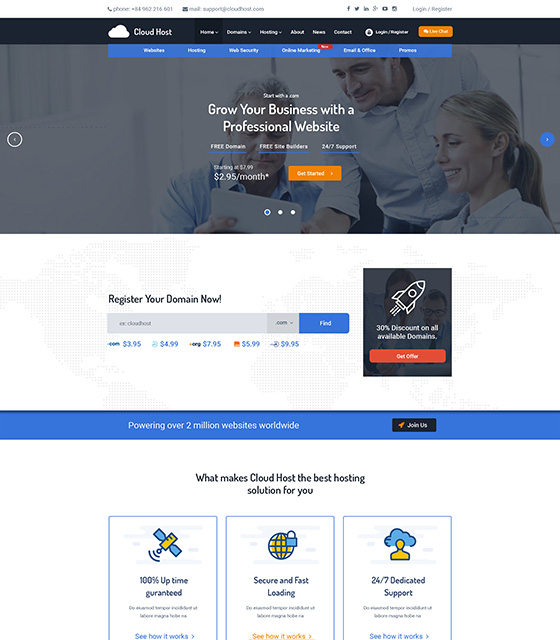This is a low-quality and small screenshot of a website. At the very top, there is a white bar featuring black text that provide contact information: "Phone: 846-922-1660" followed by an envelope icon and the text "Mail: support@cloudhost.com." Additionally, the bar includes social media icons for Facebook, Twitter, Instagram, Google+, YouTube, and Pinterest, along with a "Login/Register" option.

Below this, a black bar displays a white cloud icon accompanied by the text "CloudHost". This is followed by navigational drop-down menus labeled "Home," "Domains," "Hosting," "About," "News," "Contact," and "Login/Register." On the same bar, there is an orange button with white text that reads "Live Chat."

Further down, a blue bar with white text contains links to various services: "Websites," "Hosting," "Web Security," "Online Marketing," "Email & Office," and "Payments."

Underneath these sections, there is a photo featuring three people— all Caucasian— enthusiastically gazing at a tablet. The person on the far left is an elderly male, while the other two individuals are a middle-aged man and woman, both blond and appearing to be in their forties, all smiling widely.